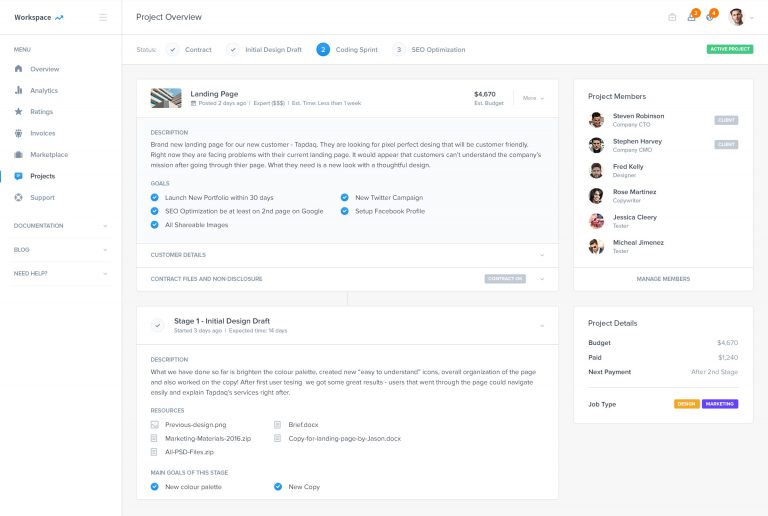This image captures a detailed screenshot of a project management and organizational dashboard. On the left sidebar, there's a blue "Workspace" button marked with a squiggly line reminiscent of a chart symbol, followed by a hamburger menu icon. This sidebar menu includes various sections such as Overview, Analytics, Ratings, Invoices, Marketplace, Projects, and Support, each accompanied by respective icons. Below these, there are three additional categories without icons: Documentation, Blog, and Need Help.

The main part of the screen prominently displays a "Project Overview" section. Here, users can see a series of tabs running horizontally across the top, labeled as Status, Contract, Initial Design Draft, Coding, Sprint, and SEO Organization. At the center is a green "Active" button indicating the current state of the project, labeled "Lending Page," with a budget allocation shown as $4,670.

To the right side of the main area, there are notifications for unanswered messages, and a list of project managers or team members' names is listed vertically. This platform appears to be highly structured, designed to facilitate the management of a building or development project through organized sections and user-friendly navigation.